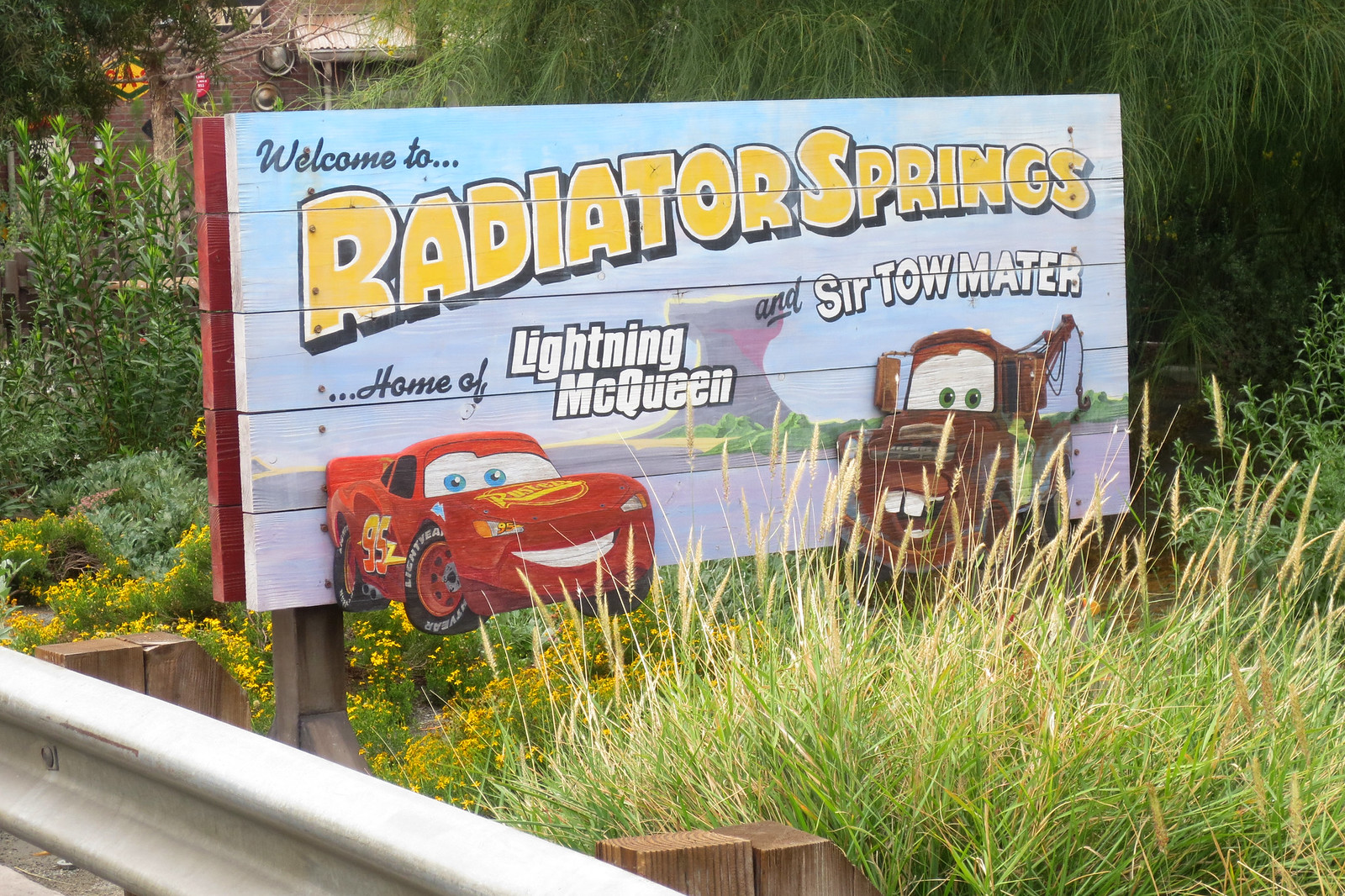In this outdoor photograph, we see a large, rectangular, wooden roadside sign welcoming drivers to Radiator Springs. The sign is centered in the image and has a light blue background. Across the top, in black script lettering, it reads "Welcome to...". Below this, in large, curved, and slightly diagonal yellow print outlined in black, it says "Radiator Springs." Beneath this text, the sign features two cartoon vehicles from the movie "Cars."

On the left, there's a vibrant red racecar with blue eyes and a wide, white, toothy smile. This is Lightning McQueen, identifiable by the text above it in white lettering outlined in black that reads "Lightning McQueen." To the right of Lightning McQueen is a tall, rusty brown tow truck, named Sir Tow Mater. The truck has brown eyes and an open mouth with distinct white buck teeth, with the text above it in black script reading "AND Sir Tow Mater."

The setting around the sign includes a grassy area in the foreground with tall reeds partially obscuring the lower part of the sign. To the left, there is a highway metal guard rail, indicating the sign's placement by the roadside. Behind the sign, there is a grassy field with a mix of green foliage, tan-colored plants, and a variety of shrubs with yellow flowers. Tall trees, possibly birches or willows, form a dense forest backdrop, adding to the lush outdoor environment. 

The photograph overall is full of vibrant colors such as red, brown, yellow, light blue, green, and tan, and it captures the whimsical charm of the "Cars" movie characters welcoming visitors to their animated hometown.